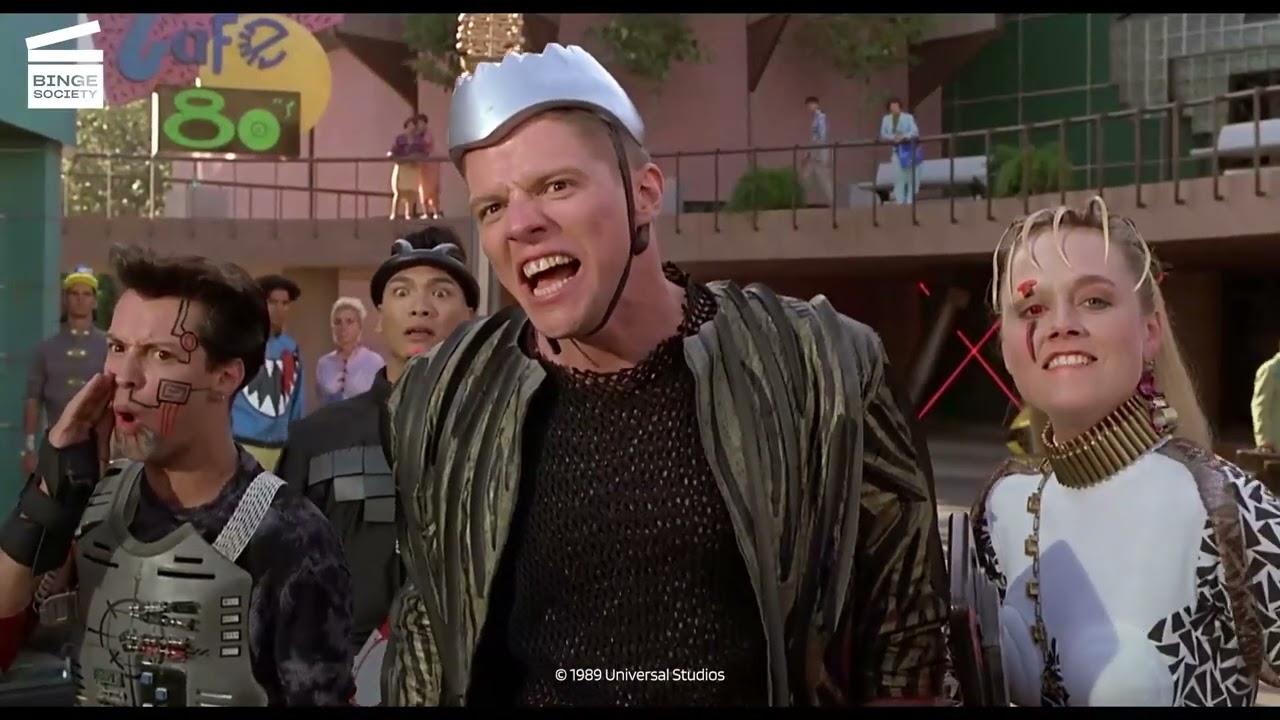The image depicts a vibrant scene, likely from a movie or a show, with characters clad in extravagant costumes. At the center stands a man wearing an olive green vest over a black mesh shirt, paired with a silver helmet that has a black strap. His expression features an open jaw. To his right, a shorter woman with blonde hair is seen wearing a white bodysuit adorned with pieces of cut glass and a striking gold headdress with spikes protruding from it. The background reveals more elaborately dressed individuals, along with a balcony filled with people. In the top left corner, "Binge Society" and "Cafe 80s" are visible, while at the bottom left, there is a "Copyright 1989 Universal Studios" label. The setting appears lively, filled with characters that look almost futuristic with elements like robotic chest plates and drawn-on circuits.